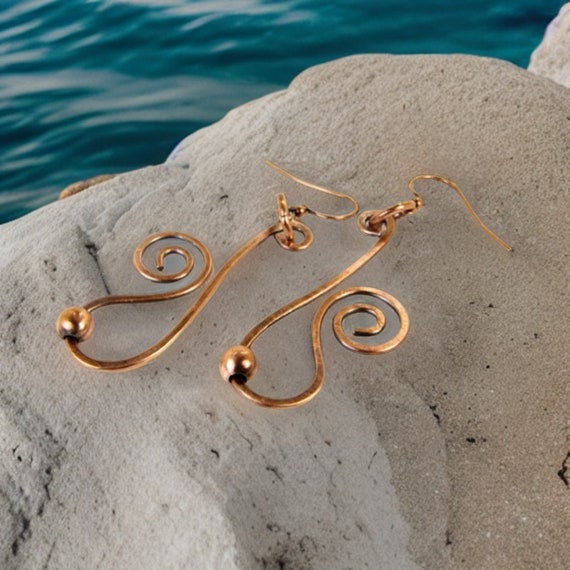This professional photograph showcases a pair of striking earrings displayed on a textured, grey rock with pockmarks, accompanied by a backdrop of serene, teal-colored water. The earrings are gold-colored, with a distinctive design that resembles the treble clef symbol from sheet music. Each earring features a flowing, curvy line that gracefully spirals into a coiled loop at the end. Adding to their elegant design, each earring includes a small golden sphere or bead near the bottom and hooks for wearing. The image is composed to highlight the beauty and intricacy of the earrings, with one earring's spiral facing left and the other's facing right, capturing their mirrored symmetry and exquisite detail. The natural setting enhances the appeal of the jewelry, making it an eye-catching and memorable display.